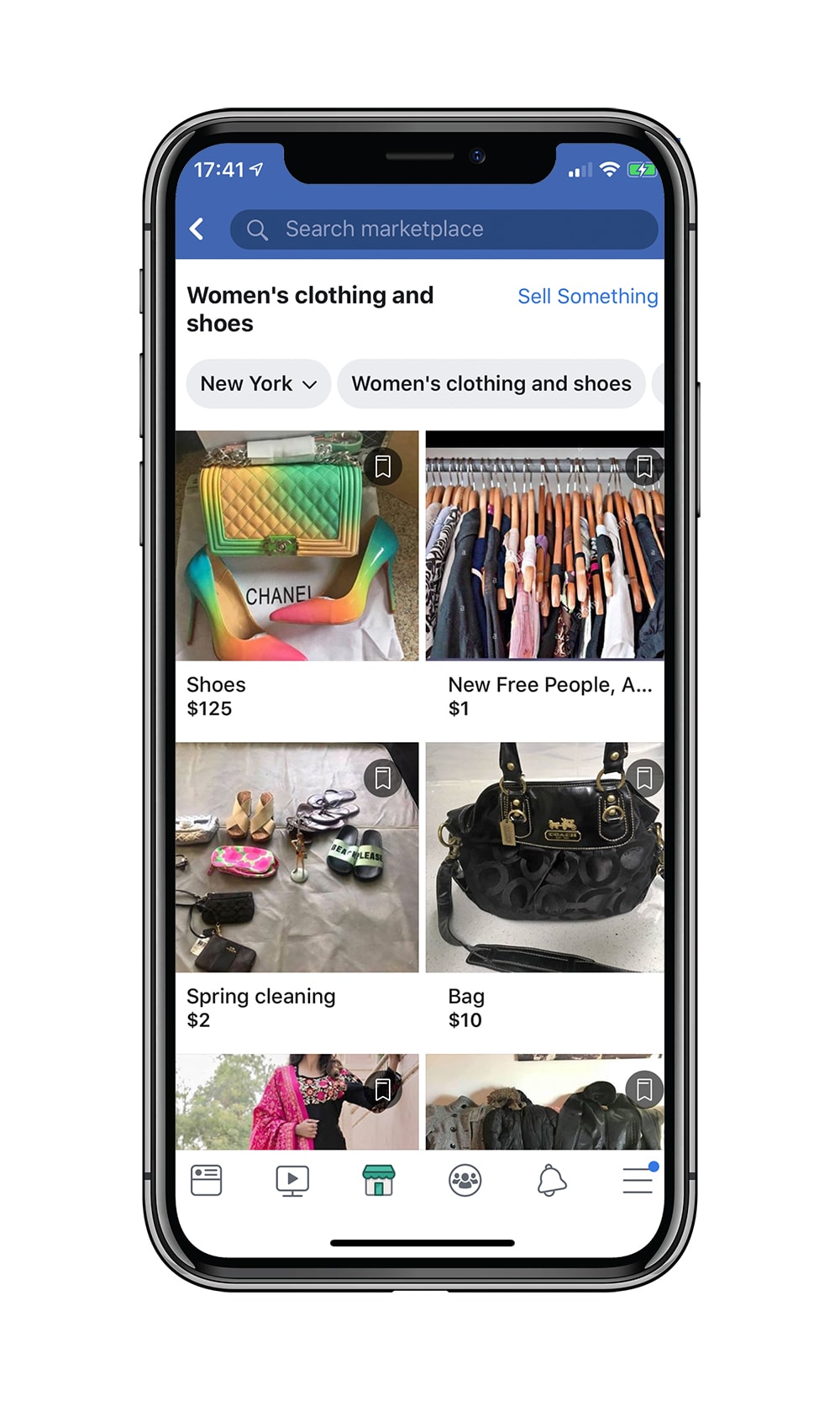The image is a detailed screenshot of a smartphone display, set against a pristine white background, giving it the appearance of a professional product image. The screenshot prominently features the Facebook Marketplace interface. The top of the screen displays the "Search Marketplace" bar in Facebook's signature dark blue color, contrasting with the predominantly white background below.

In the focal area of the screenshot, six images of various products being sold on Facebook Marketplace are visible, though only four are clearly identifiable. 

- At the top left, a vibrant pair of rainbow-colored heels priced at $125 is labeled as "Shoes."
- At the top right, a listing titled "New Free People" shows a product priced at $1, potentially hinting at free or very low-cost clothing items.
- The bottom left corner features a post labeled "Spring Cleaning" with a price tag of $2, depicting a variety of clothes and miscellaneous items spread out on a bed.
- In the bottom right, a simple black purse is listed under the name "Bag" and is available for $10.

The bottom two listings are partially visible, with their names and prices obscured. The overall clarity and arrangement suggest that the screenshot might have been digitally placed onto the phone image to create the illusion of an active phone display.